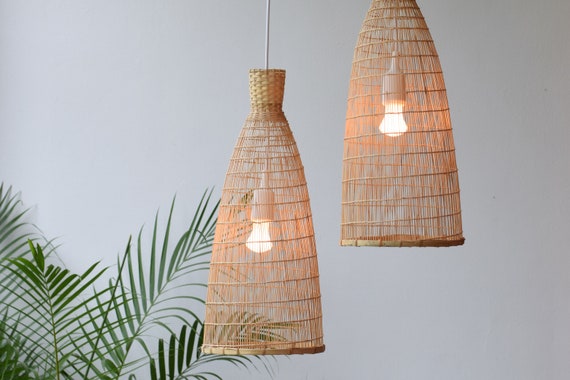The image is an indoor scene featuring two dome-shaped wicker lampshades hanging from the ceiling, giving off a tiki lounge vibe. The left lamp is suspended from a visible wire, while the right lamp hangs higher, obscuring its fixture. Both lampshades encase lit light bulbs. In the background, a bluish-gray wall serves as a subtle, neutral backdrop. On the left side of the image, there is a healthy, lush green fern with tall leaves spreading in various directions, adding a touch of nature to the setting. The top of the plant is visible, but the pot is out of frame. The overall ambiance is cozy and inviting, suggesting a well-decorated home interior.